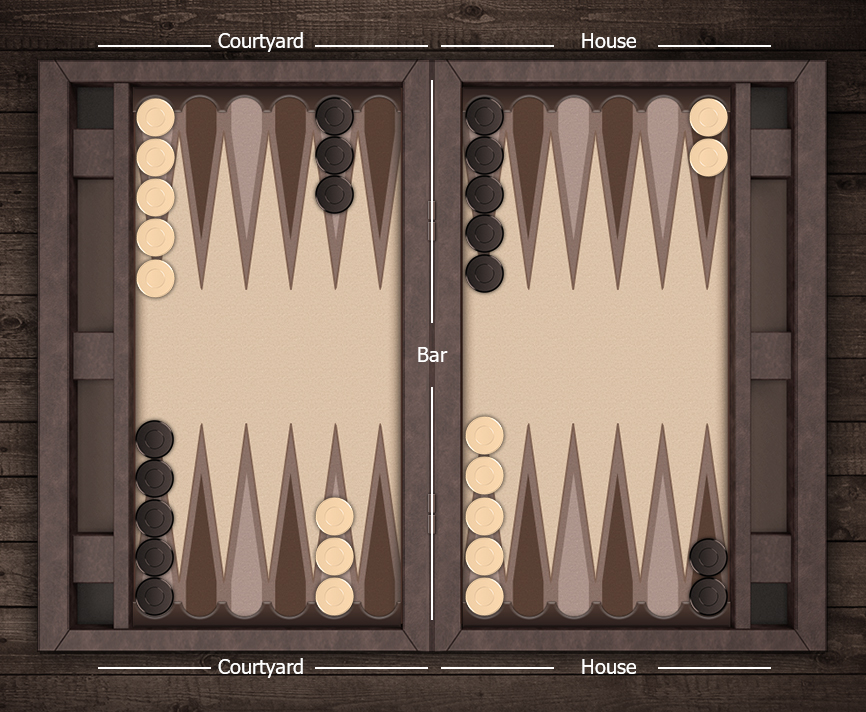The image depicts a backgammon board, prominently featuring its recognizable elements and setup. The board is laid out with alternating light and dark circular tokens—some of a white or cream color, and others dark brown or nearly black. Surrounding the playing area is a darker brown wooden border. Overlaying the intricate tan, gray, and brown board pattern is white lettering: the word "Courtyard" appears at the top left and bottom left, while "House" is positioned at the top right and bottom right; the term "Bar" runs through the center of the board, demarcating the two halves. The backgammon set is placed on a dark brown wooden surface, where the wood grain is visible, possibly indicating a table or flooring. The tokens are arranged in their starting positions, with specific groups (five dark in the top left corner, five light below them; similar setups on the opposite side and corners) as a typical opening setup for the game.